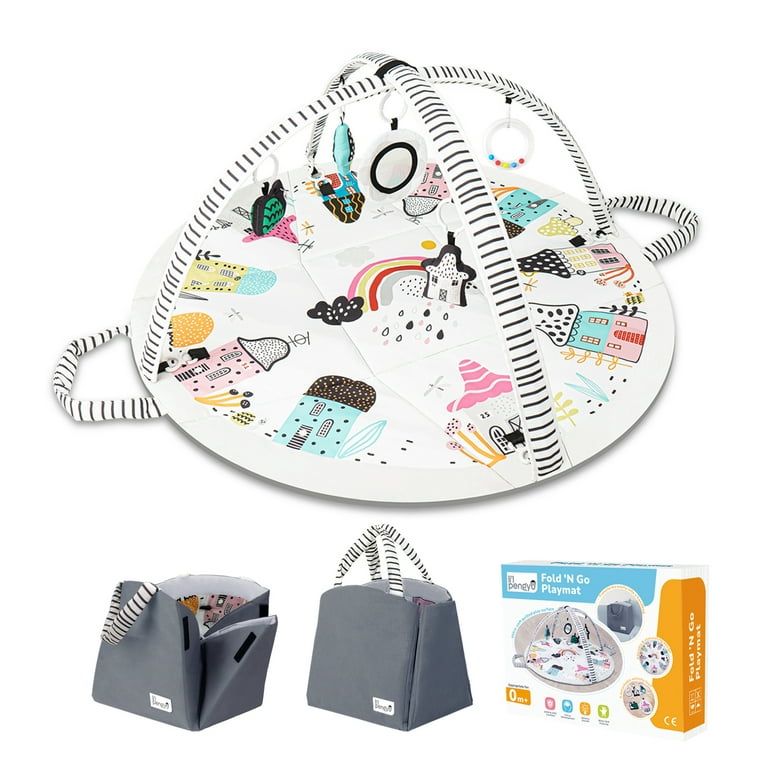The image features a beautifully detailed baby playmat set against a plain white background with no visible borders. The main attraction at the top of the image is a round, white playmat adorned with charming designs such as colorful houses, a vibrant rainbow, and various flowers, arranged in a way that would delight any child. Black-and-white striped fabric arches cross over the playmat, with adorable toys like a turtle, a fish, and dotted rattles hanging down for endless play.

Beneath the playmat, a sequence of three images showcases the product's versatility. On the left, the playmat is neatly folded up, showing its solid gray exterior with zebra-striped handles. The center image presents the playmat fully closed, resembling a chic handbag with its handles pointing upward. To the right, a box labeled "Fold & Go Playmat" provides a preview of the items seen above, encapsulating the convenience and style of this versatile baby playset.